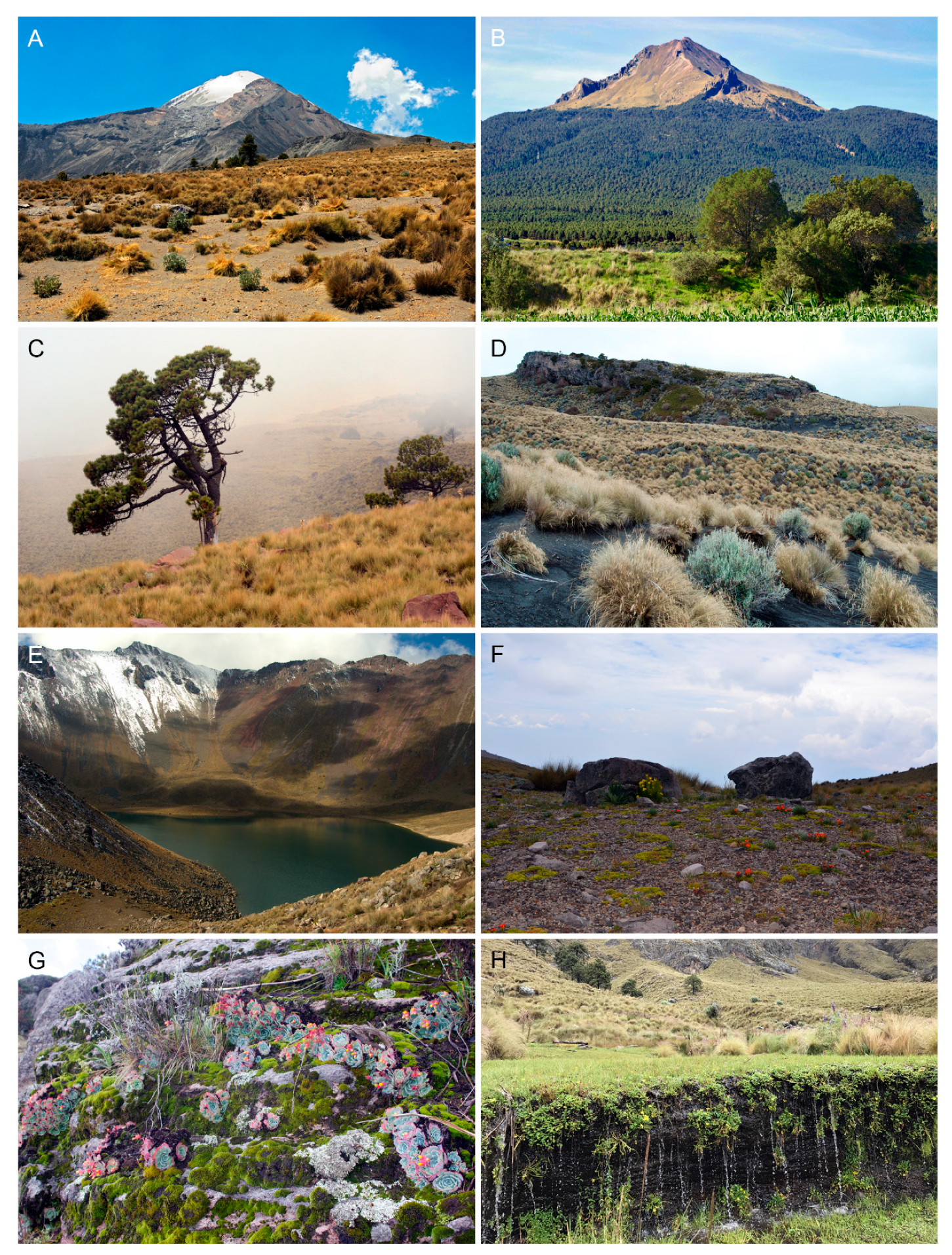The series of eight landscape photographs labeled from Exhibit A to Exhibit H captures a diverse range of natural scenes, displayed in a grid format with two images per row. 

- Exhibit A presents a desert landscape featuring a tumbleweed-strewn foreground with a rugged mountain range in the background. 
- Exhibit B showcases a lush forested mountain range, displaying a verdant expanse of greenery.
- Exhibit C depicts a desolate scene with a cliff edge adorned with a solitary barren tree and dry, brown grass.
- Exhibit D highlights a rocky terrain with scattered bushes and shrubs growing at the base of a plateau.
- Exhibit E offers a tranquil view of a small lake encircled by formidable mountains and rocky outcrops.
- Exhibit F focuses on a flat, open landscape with a pair of prominent rocks standing amidst sparse vegetation.
- Exhibit G features an intriguing sight of rocks seemingly blooming with various small flowers, adding a burst of color.
- Exhibit H, similar to G, shows rocky ground with delicate flowers or possible fungal growth, intricate in detail.

All of these photographs collectively depict diverse and unique natural environments, ranging from arid deserts and lush forests to rocky plateaus and serene lakes.